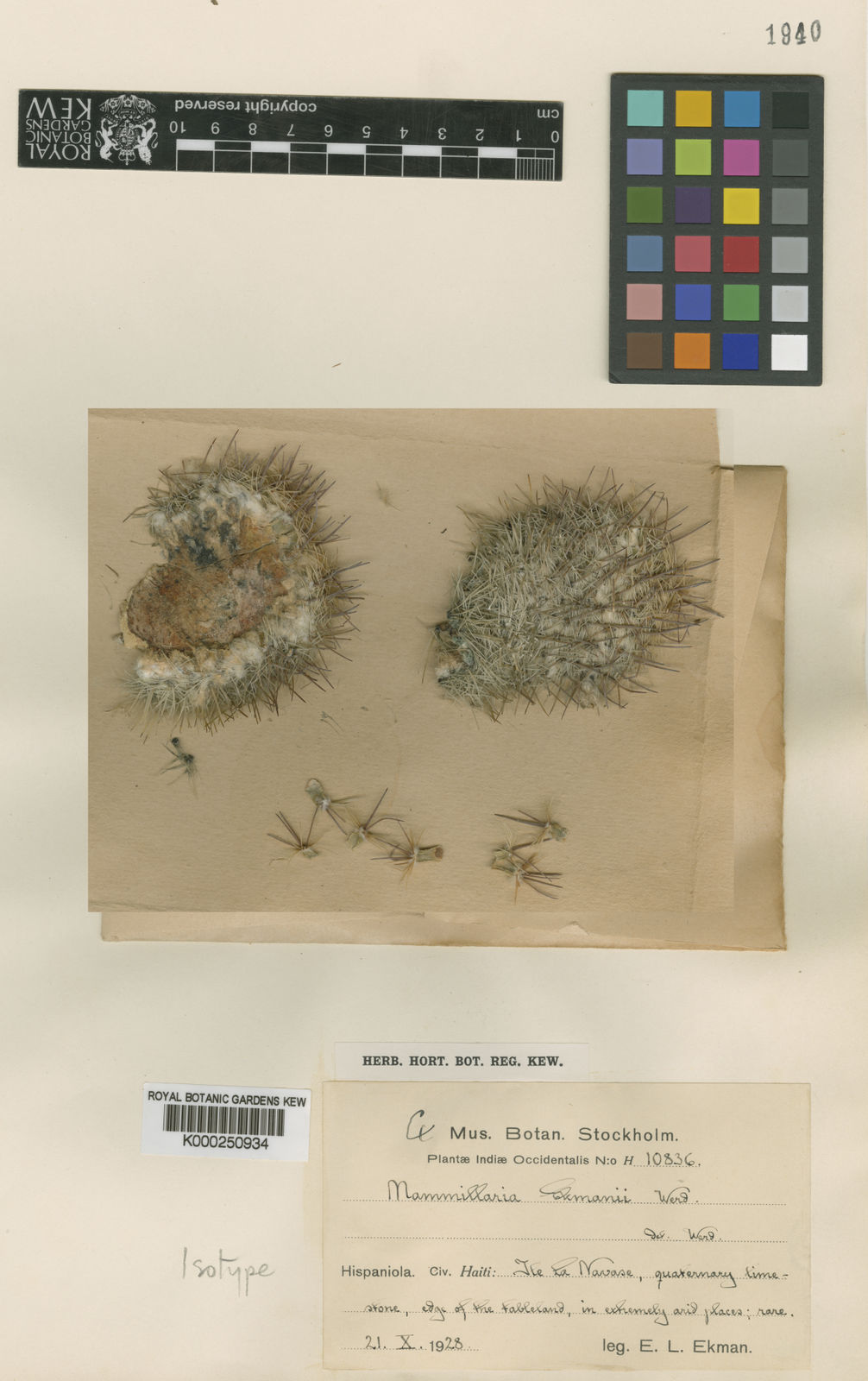The photograph, in portrait orientation, showcases a detailed children's art project on an aged, light tan parchment paper, teeming with an array of elements. Centered are two overlapping pieces of darker tan paper, adorned with what appears to be seeds and seed pods. One of the clusters, on the left, intriguingly resembles the Rolling Stones' tongue logo with a pinkish “tongue” area, encircled by spiky, twig-like substances. The other cluster mostly comprises light white and brown twiggy materials, suggesting a naturalistic theme.

Above the central composition, on the top left, is an inverted black strip of paper with reversed text, reading "Royal Botanic Gardens" and a shield logo visible. To its right is a vertically oriented, multicolored rectangle resembling a color palette with about 24 different hues, ranging from various yellows, oranges, reds, whites, and blacks. At the very top, a stamp marked "1940" indicates the historical context of the piece.

Towards the bottom, there is a typewritten certificate strip labeled "MUS. BOTAN. Stockholm," possibly denoting a botanical collection, alongside handwriting filling in additional lines. Below that, on the left, a barcode reads "Royal Botanic Gardens" with "New" visible and, beneath that, the handwritten word "Isotype" in pencil. The project's elements are meticulously arranged on the textured, cream-colored paper, blending realism with representational art styles.